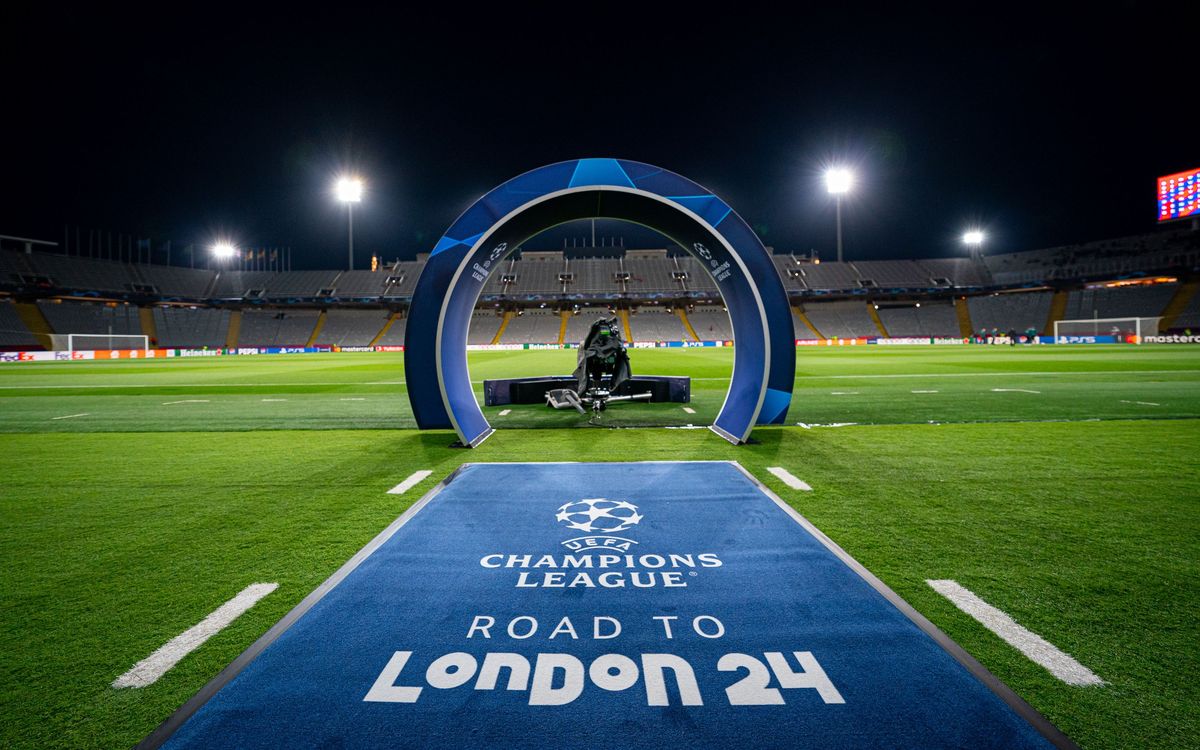The image depicts a large soccer stadium at night, illuminated by stadium lights. The central feature is a lush green soccer field, surrounded by silver bleachers. In the foreground, there is a blue carpet leading up to a circular archway, which seems to be an entrance or tunnel for players. The blue carpet bears the inscription "UEFA Champions League Road to London 24". On the field, there are soccer nets visible on both the left and right sides, indicative of an upcoming match. The scene is devoid of spectators and players, making the stadium appear eerily empty. A lit sign is partially visible in the upper right-hand corner, hinting at stadium signage or advertisements.